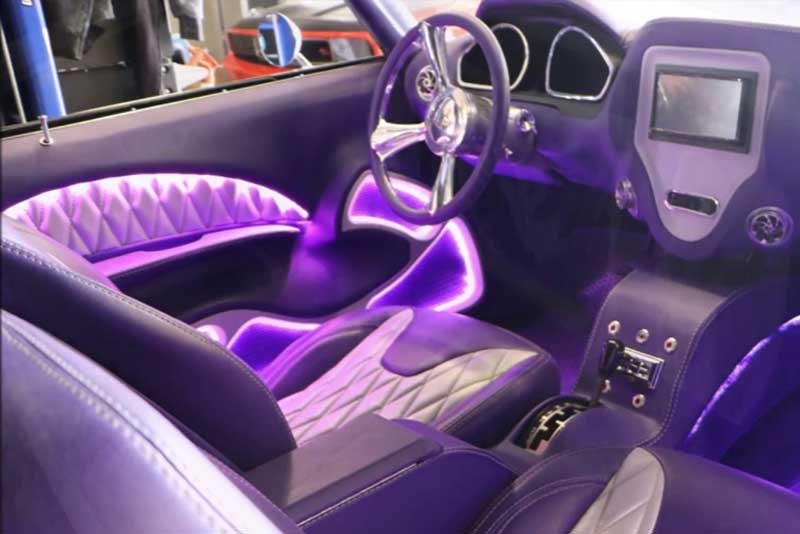The image showcases the interior of a highly stylized car, predominantly bathed in a striking purple hue that gives it a luxurious and unique appearance. The dashboard, steering wheel, middle console, and plush, diamond-patterned seats are all adorned in this rich purple color. Notably, the steering wheel features a silver center. The door panels are quilted with the same diamond pattern found on the seats, enhancing the sense of continuity and design. The driver's door includes a push button for locking and unlocking. Central to the dashboard is a screen flanked by two knobs, below which resides a vertical gear shift lever and what appears to be a radio. Outside the car window, another vehicle, colored orange, can be seen, along with the interior of a garage. The photo, horizontal and rectangular in shape, is illuminated with a purple tint that further accentuates the opulent vibe of the car's interior, signifying a high-end, well-cushioned design.